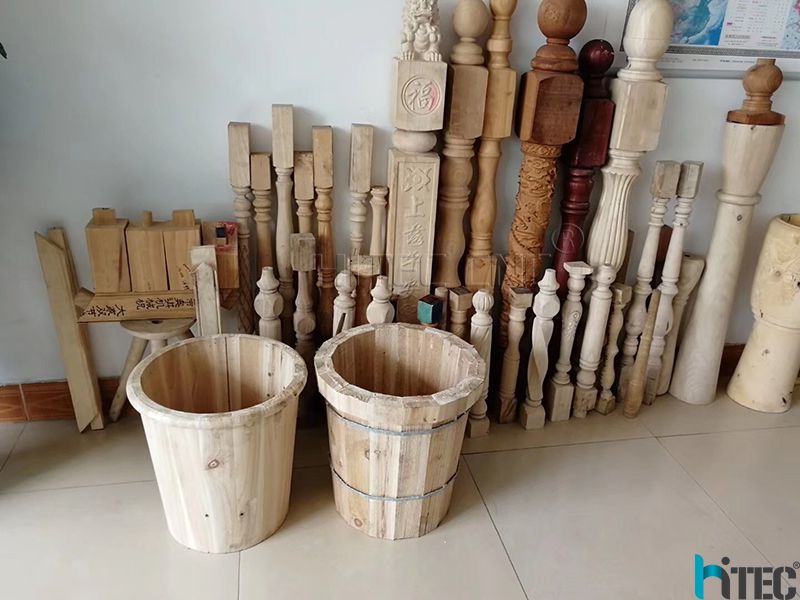The photograph captures a detailed scene from a woodworking exhibit or workshop, likely in an Asian-speaking country, as suggested by the visible Asian script and a map that appears to show China on the white-tiled wall. In the foreground, two banded, intricately carved wooden buckets stand, resembling small planter boxes. Behind them, a diverse collection of banisters made from various types of wood occupies the background. These banisters, in heights ranging from small to large, showcase a mix of finishes—stained, painted, and unfinished. Many of them exhibit detailed carvings and spiral patterns, with one particularly notable banister featuring an ornate dragon on top. The workshop's floor is tiled, with a wooden trim at the base of the wall. A logo, "HITECH" with a copyright symbol, is present in the lower right corner, reinforcing a sense of craftsmanship and pride in the displayed woodwork.